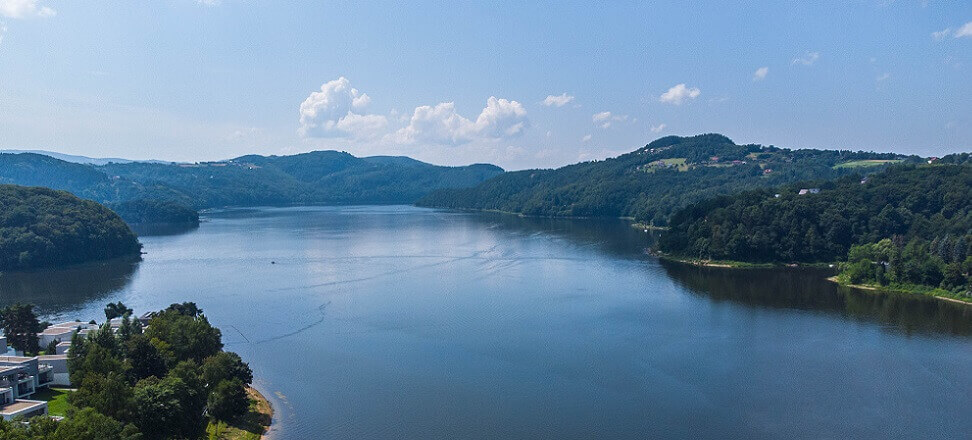This is a stunning color photograph, possibly taken from a slightly elevated angle, featuring a wide, expansive lake on a clear, sunny day. The top third of the wide, rectangular image captures a beautiful blue sky adorned with a few white, wispy clouds. The lake, situated at the very center, mirrors this serene sky, enhancing the tranquility of the scene. Encircling the lake are mountains and hills covered in lush green trees, with some particularly high hills adding depth to the background. Along the right-hand side of the mountains and on the left side's jutting land, there are some gray and white structures, possibly homes or buildings, partially obscured by the dense greenery. The foreground reveals a grassy shoreline lined with trees, where more large structures can be seen. The overall scene is devoid of any human presence, allowing the natural beauty and reflection in the clear water to take center stage.